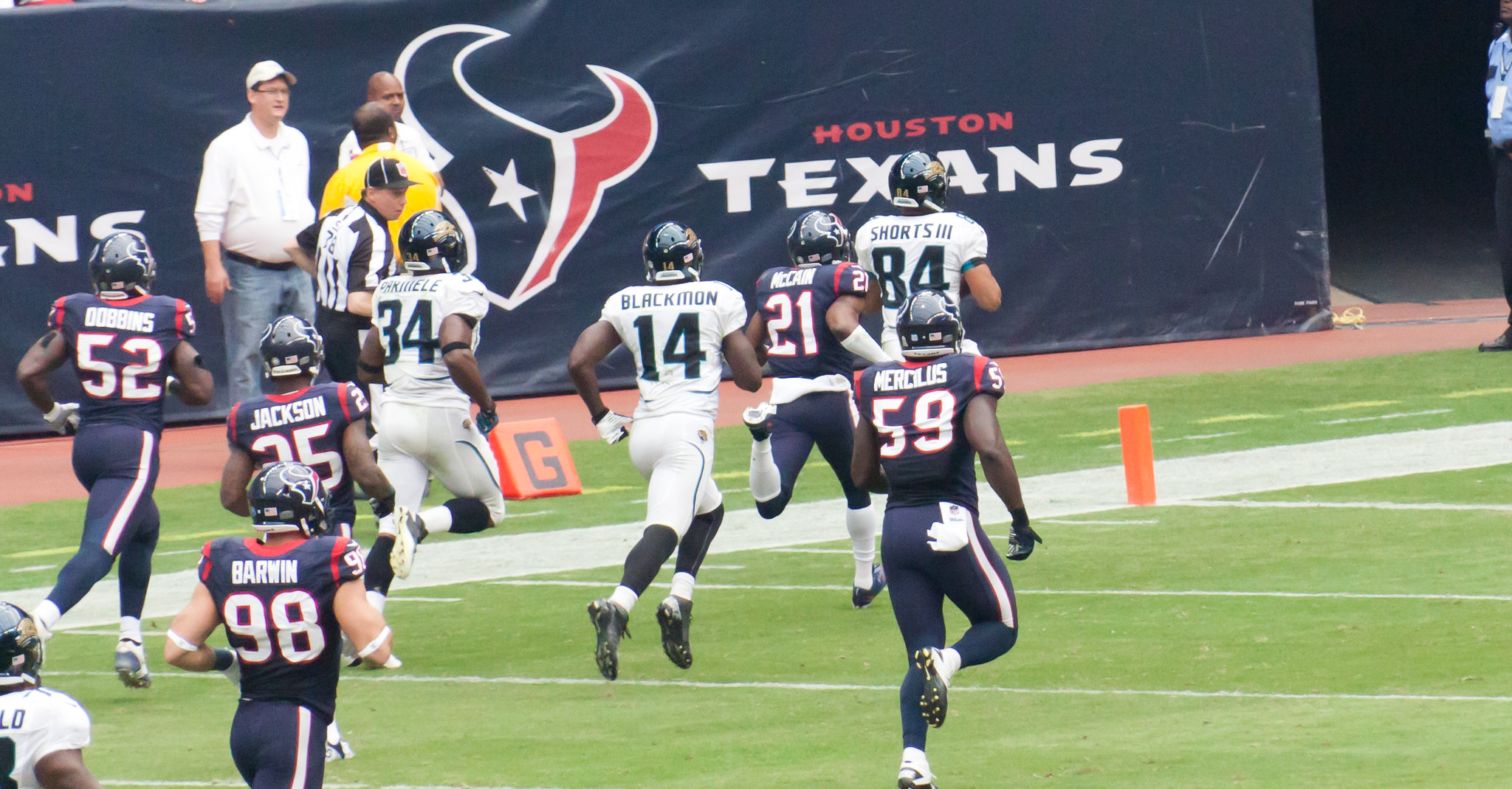This image captures a dynamic play during an NFL football game featuring the Houston Texans and the Jacksonville Jaguars. The photograph, possibly taken with a telephoto lens or from a television broadcast, offers a close-up look at several players sprinting toward the end zone. The main action centers around the likely ball carrier, number 84, pursued closely by several players including number 21. The Texans are donning their dark blue jerseys with white numbers and red trim, while the Jaguars are in their white uniforms with dark blue or black numbers. The green football field, marked by white lines and orange pylons indicating the beginning of the end zone, sets the stage for this intense moment. On the sidelines, there is a noticeable dirt track bordering the turf and a prominent dark blue backdrop displaying the Houston Texans logo. Additionally, a referee and coaching staff members are visible, adding to the authentic game-day atmosphere.